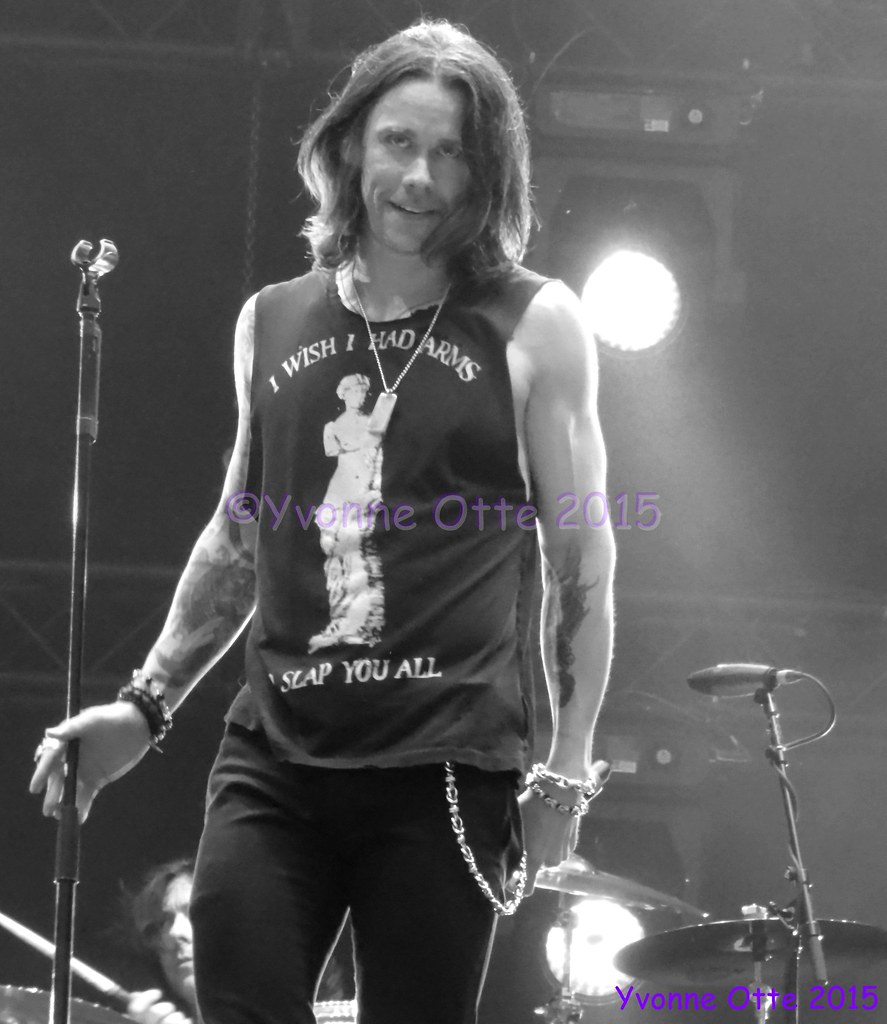This black-and-white vertical photograph captures an intense stage performance. At the center, an entertainer stands gripping a microphone, bathed in contrasting shades of black, white, and gray. He wears tight jeans with a watch chain dangling from the loops and a striking sleeveless shirt emblazoned with the phrase, "I wish I had arms to slap you all," featuring the iconic armless Venus de Milo statue. His arms are adorned with bracelets on both wrists. Behind him, partially visible, is a drummer seated at a drum set, drumsticks poised and ready, signifying the musical nature of the scene. The stage is set indoors, under dim lighting that accentuates the dramatic ambiance. Additional stage equipment and lights are faintly discernible in the background, while the photograph is credited to Yvonne Ott, 2015.